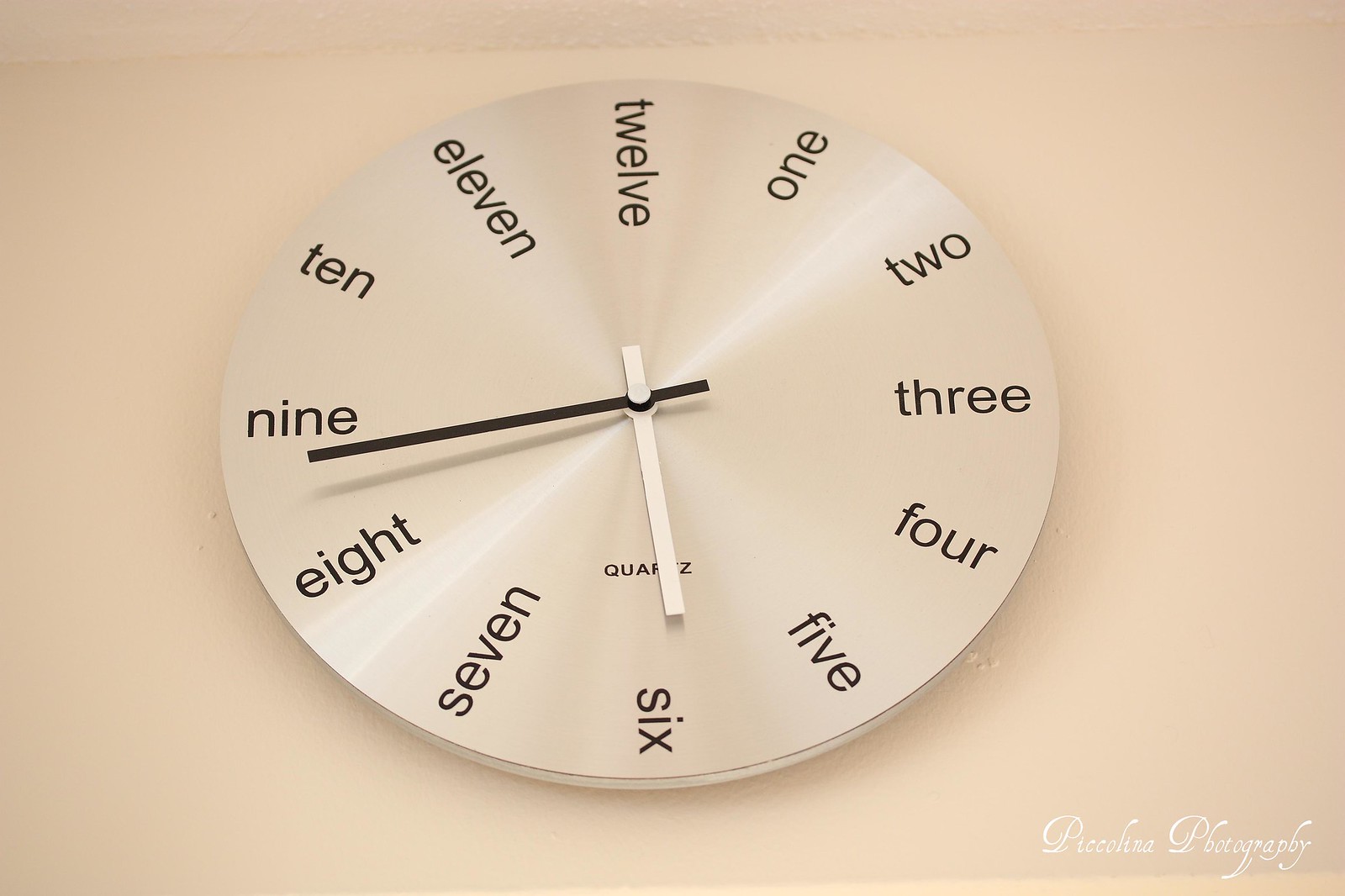The image depicts a modern analog clock mounted on a cream-colored wall, blending subtly with the slightly off-white circular face of the clock. The clock features a unique design where the numerals are replaced with lowercase black text spelling out the numbers from 'one' to 'twelve'. The minute hand, colored in black, is near the 'nine' while the white hour hand points just above 'six', indicating a time close to 6:45. Near the bottom of the clock face, the text 'HORTS' is displayed, seemingly representative of the clock's brand. In the bottom right corner of the image, there's faint white text that reads "Pecolina Photography." The clock's minimalist design, with its worded numerals and contrasting hand colors, stands out against the slightly textured background.